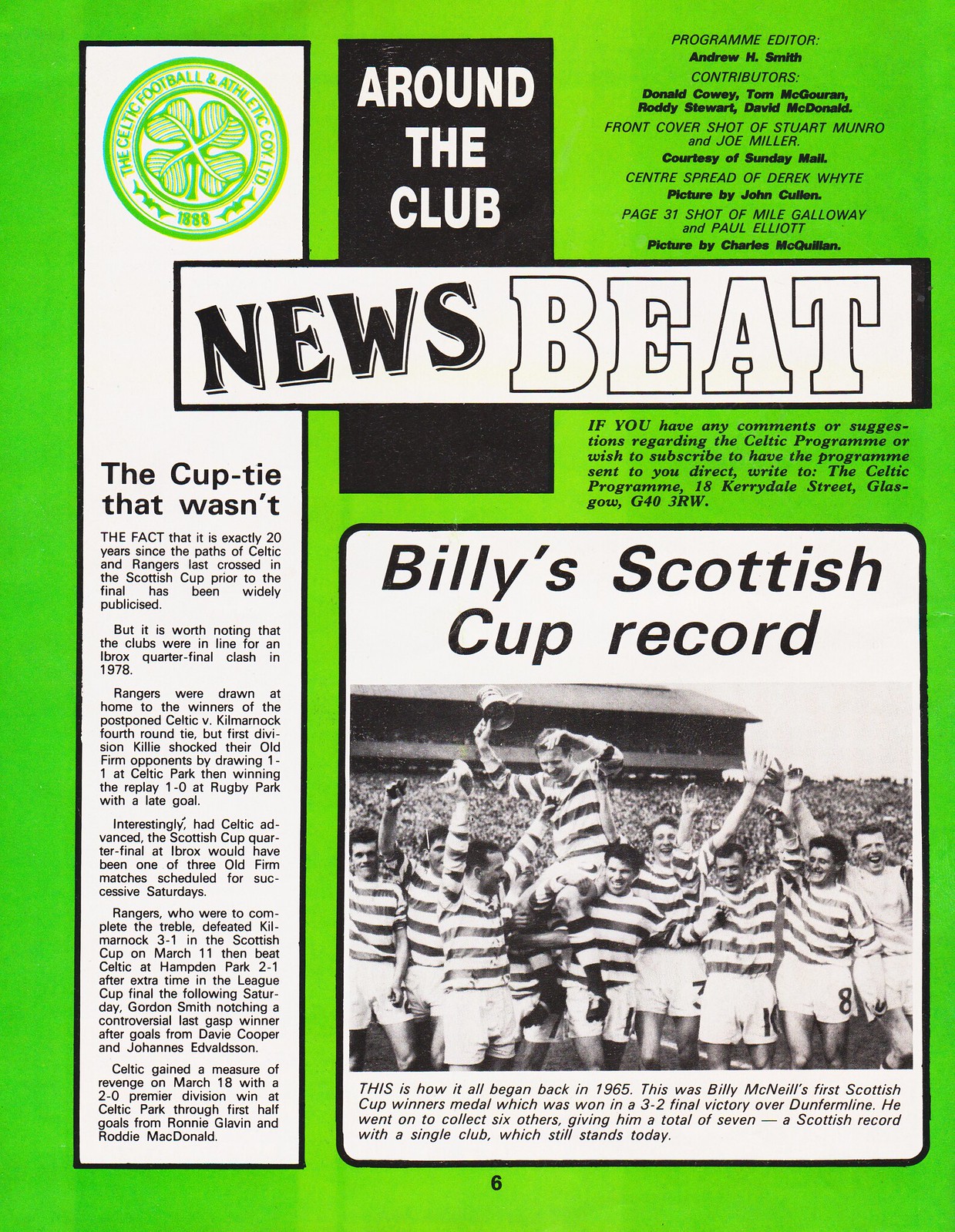The image showcases a scan of a football program's page, predominantly page six, as indicated by the black number six on a bright green background at the very bottom. The page is segmented into various text sections and images. One prominent section on the lower right, enclosed in a rounded square, is titled "Billy's Scottish Cup Record." Accompanying this section is a caption: "This is how it all began back in 1960, possibly 1965."

A striking black-and-white photograph occupies a significant portion of the page, featuring a jubilant football team. The players are clad in horizontally striped shirts paired with plain white shorts, with visible numbers on the shorts. One player, elevated on the shoulders of his teammates, adds to the celebratory atmosphere, while a grandstand filled with spectators forms the backdrop.

At the top of the page, the titles "Newsbeat" and "Around the Club" introduce smaller sections of text detailing contributions from the Program Editor and various authors, along with a feature titled "The Cup Tie that wasn't." Additionally, the emblem of Celtic Football and Athletic Co. Ltd., in green, is prominently displayed in the left-hand corner, reinforcing the page's association with the football club.